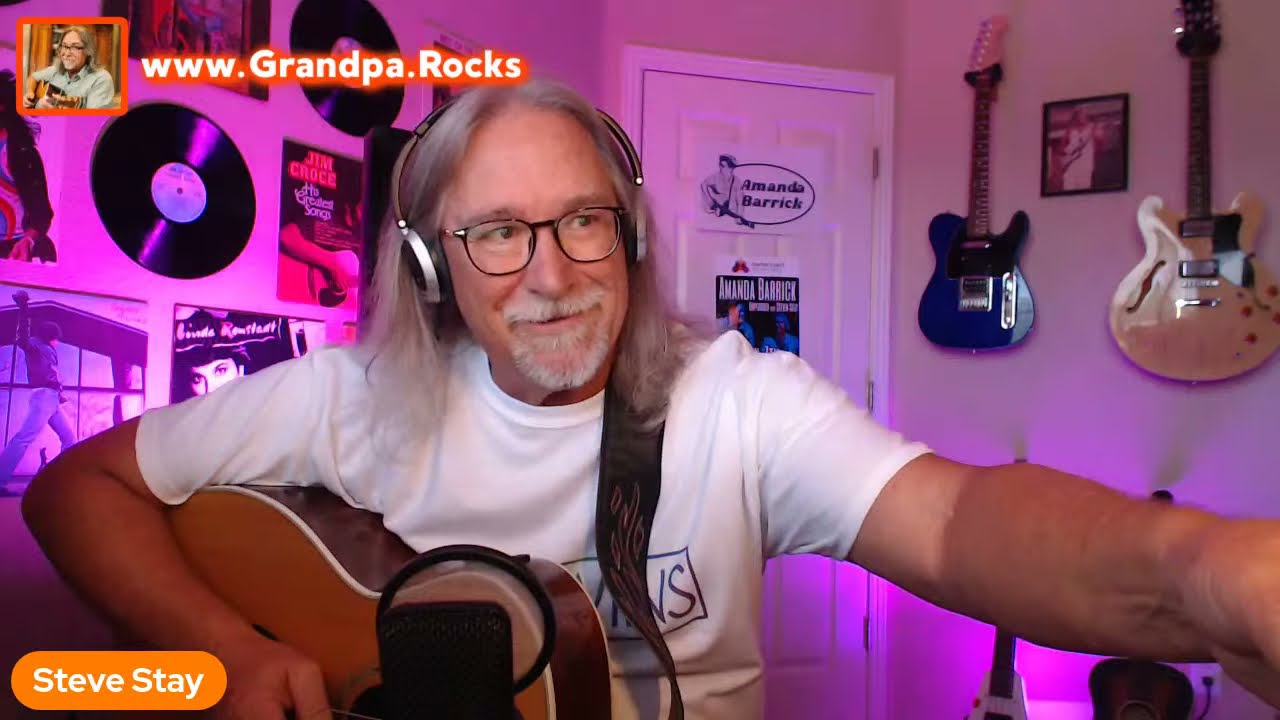This color photograph shows an older man with long gray hair, a white beard, and a little ponytail draped over his shoulder. He is seated in a bedroom, wearing black eyeglasses, silver headphones, and a white t-shirt with a black logo on the front. The man is holding an acoustic guitar characterized by light and dark brown tones, which rests in his lap with a strap slung over his shoulder and neck. He uses his right hand, extended outwards, possibly to adjust the camera for a selfie video, while his left hand holds the guitar against his body.

The background features a white door with two pieces of paper attached; the upper one depicts a figure with a guitar and an unreadable text bubble, and the lower one is a colored picture with text against a blue background. Additionally, the room includes various vinyl records, album covers, and guitars—specifically, a blue and a brown guitar hanging on the wall and two more on the ground illuminated by a purplish light, alongside a small photo in between.

In the lower left corner, there is an orange bullet-shaped text box with "Steve Stay" in white upper and lowercase letters. The top left corner displays a small photograph of the man in an orange-bordered inset, accompanied by the website URL "www.grandpa.rocks" in white text with an orange drop shadow. The overall style of the image is a detailed, photo-realistic screenshot from a video.